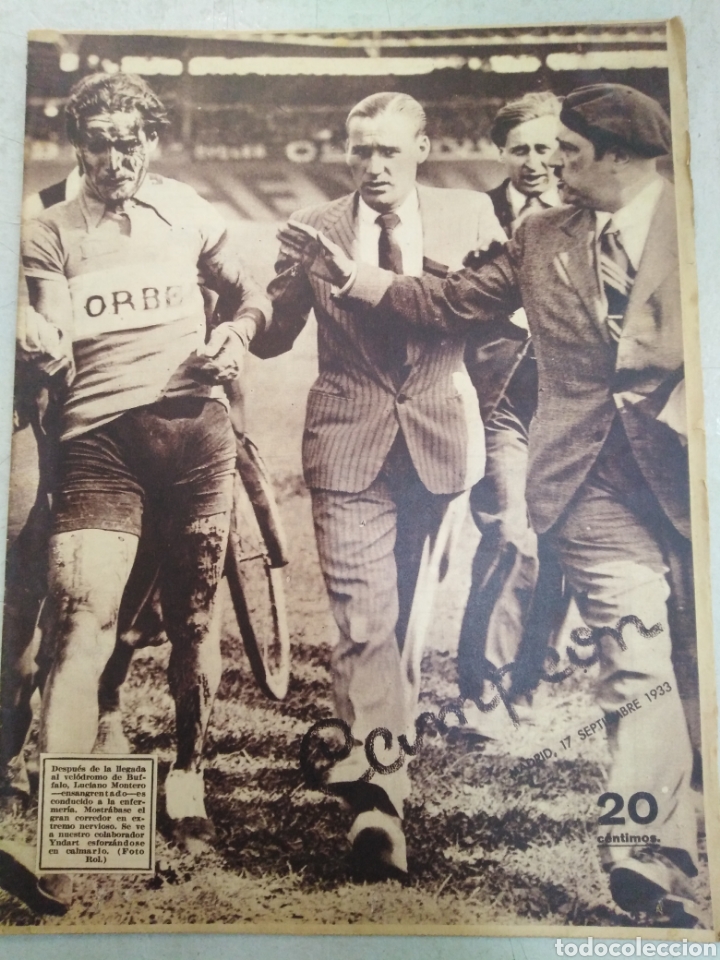The vintage black-and-white photograph, likely taken during a sports event on September 17, 1933, in Madrid, captures a striking scene set within a grassy stadium field. At the forefront stands a mud-covered cyclist dressed in a white jersey adorned with the letters "ORB", alongside snug-fitting brown shorts. His face is distinctly marked with dirt. To the right, two well-dressed men accompany him. The man closest to the cyclist wears a beret, a black tie, and a pinstripe suit, his hand resting on the cyclist's elbow, while a man in a plain suit with a brown tie follows slightly behind. In the backdrop, a bicycle is partially visible, hinting at the nature of the event. The poster includes a signature, potentially reading "C-C-A-M-P-E-O-N," with the numbers "20" and the word "AMPIMOS" inscribed below, along with additional text in a language that remains unspecified. The backdrop and visible crowd enhance the vintage ambiance of this unique sporting moment.